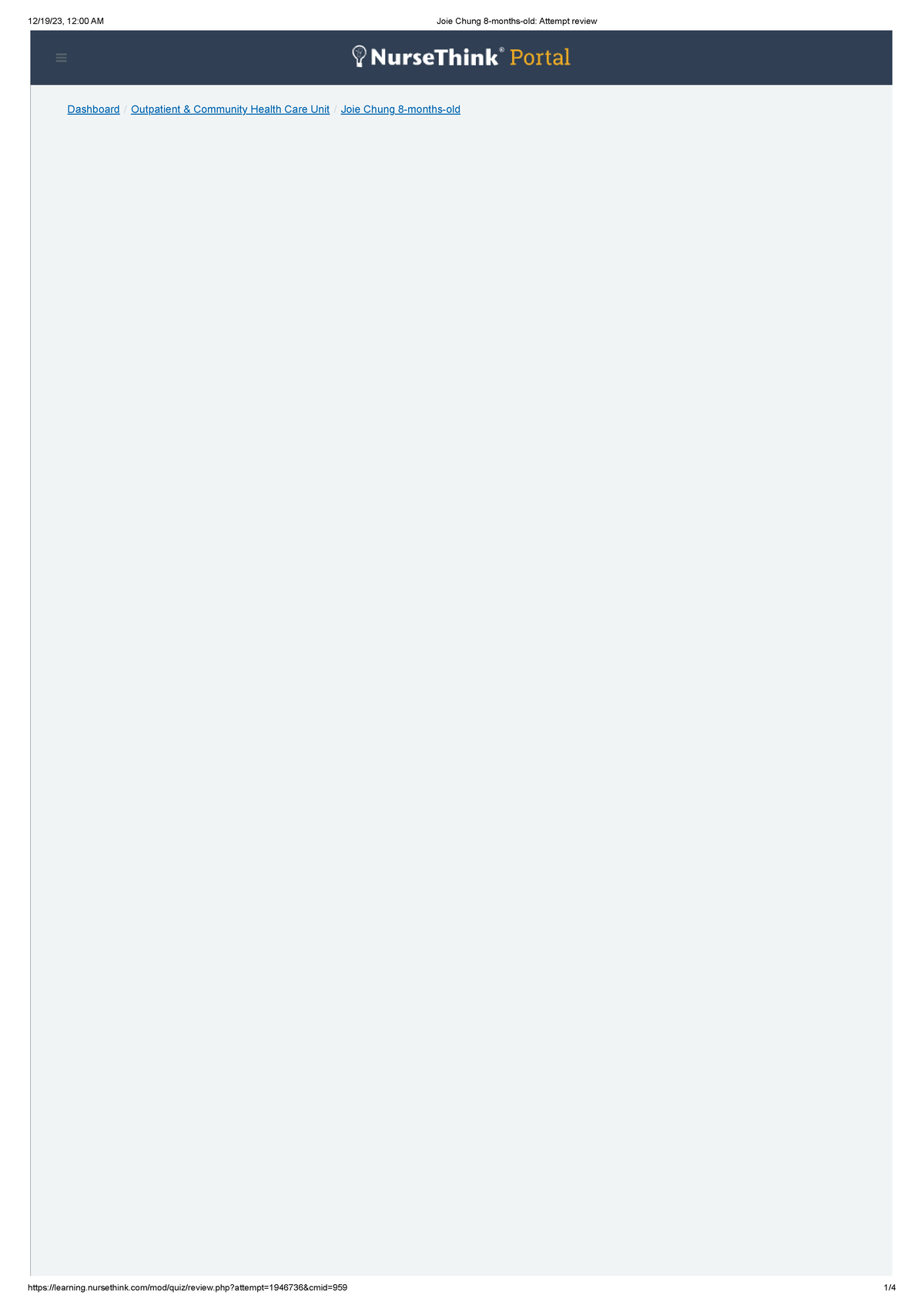The image portrays an open webpage titled "NurseThink Portal," prominently displayed at the very top. Directly below the title, there are three small, blue, underlined links, one of which is labeled "Dashboard." In the top left-hand corner, there's an indication of the date and time, but the text is extremely small and unreadable. The central area of the page features a large, light gray, empty space, dominating the middle of the image without any visible content. At the very bottom left-hand corner, there is a small black text, which is similarly unreadable, next to a logo that resembles a light bulb. The entire setup suggests that this image captures an online portal interface, specifically known as "NurseLink." The central empty space likely indicates content that has yet to be loaded or displayed.